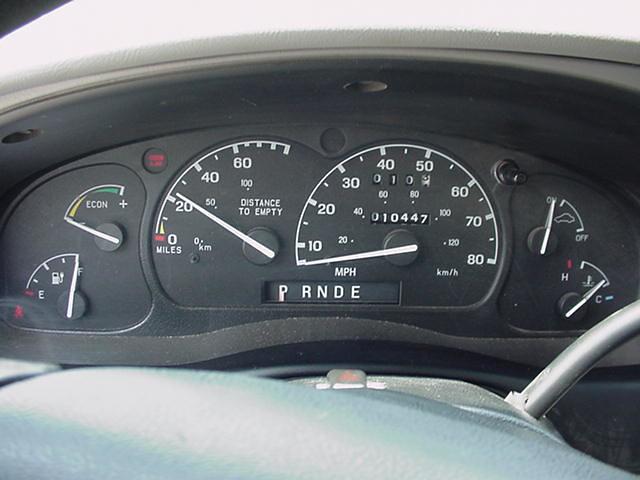The image depicts the dashboard of an automobile, showcasing an array of gauges designed for the driver's information. The dashboard and steering column share a gray or silver hue, providing a sleek and cohesive look. On the lower right corner of the image, a portion of the gear shift is visible. The emergency flasher button is centrally located at the bottom of the dashboard.

The focal point of the dashboard is a black-faced gauge display featuring two prominent gauges at its center. These gauges include white needle indicators, displaying crucial driving information. The left gauge provides details on the distance to empty, indicating just over 20 kilometers until the gas tank is empty. The central gauge combines an odometer and speedometer, with a push-button reset for the odometer. Below the speedometer, the drive indicator shows the vehicle is currently in park (P), with other gear positions (R, N, D, E) also visible.

To the left of the main gauges, an additional display labeled "econ" with plus and minus signs possibly represents battery status. Beneath this, a separate fuel gauge confirms that the gas tank is full. On the far right, two smaller gauges monitor the vehicle's radiator and water temperature (hot and cold indicators). Above these, an unrecognized symbol featuring a car outline with an on-off label is present.